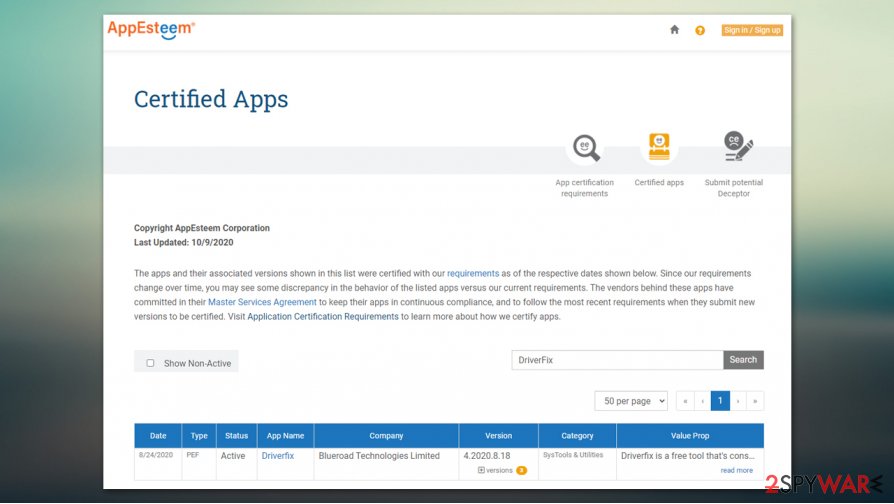The image, captured in landscape mode, appears to be a screenshot from a laptop. The background transitions from a light gradient at the top, characterized by light greens and yellows, to a darker spectrum towards the bottom, featuring deeper blues and greens. In the bottom right-hand corner, there is stylized text reading "to SPY WAR E," where "to" is in red with a preceding line, "SPY" is in black, "WAR" is in red, and "E" resembles a zigzagged Sigma symbol in black.

In the forefront, a white card is prominently displayed:

- The upper left corner of the card features the "App Esteem" logo.
- The upper right corner contains three icons: a house, a question mark, and an orange button labeled "Sign In" and "Sign Up."
- The next row contains the text "Certified Apps" in blue font.
- Below that, there is a gray background section with several elements:
  - On the right side, it states "App Certification Requirements."
  - There is a search feature to find certified apps.
  - A section that looks like a Rolodex is present, though its exact function is unclear.
  - An option to "Submit Potential Deceptor" sits at the top.

The subsequent row includes "Copyright App Esteem Corporation. Last updated October 9th, 2020."

In the bottom left-hand corner, a listing reads: "Driver Fix, Blue Road Technologies Limited," presumably indicating the app name and the certifying company.